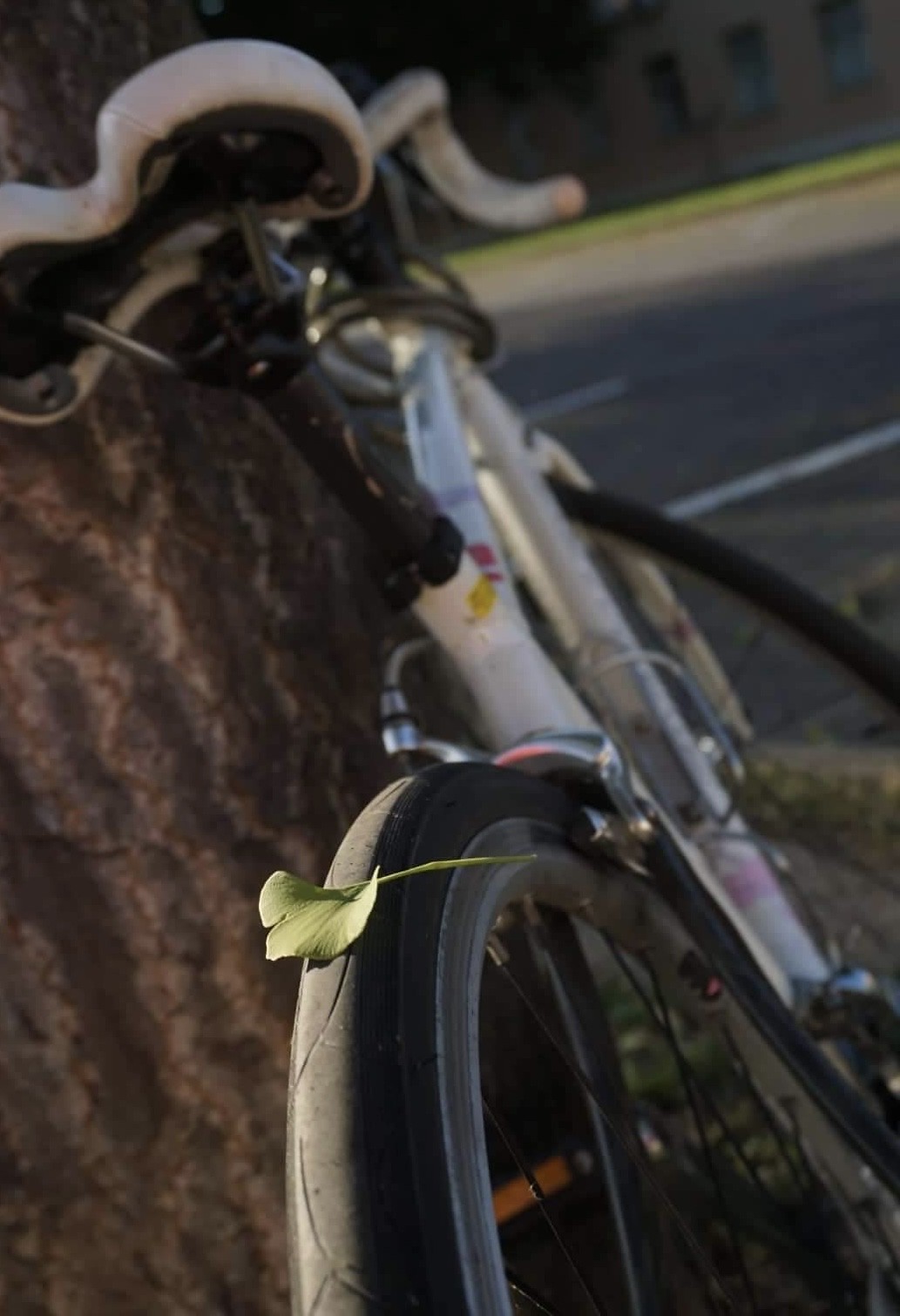The photograph captures a white single-speed road bike leaning against a brown tree, viewed predominantly from the rear. The tree’s trunk is positioned on the left side of the vertical image, extending off the frame at both the top and bottom left corners. The bicycle features a white saddle and curved white handlebars, which are prominent near the top center of the image. The rear tire, which is prominently displayed in the foreground, has a single green leaf resting on it and no tread. The bike appears to have a cable lock wrapped around its frame and a rear brake installed. The front tire is turned, extending to the right and downward out of the frame. In the background, there is a road with white markings and a patch of green grass leading to a building with visible windows in the top right corner. The overall composition emphasizes the bicycle's position against the tree with clear details of its frame and accessories.